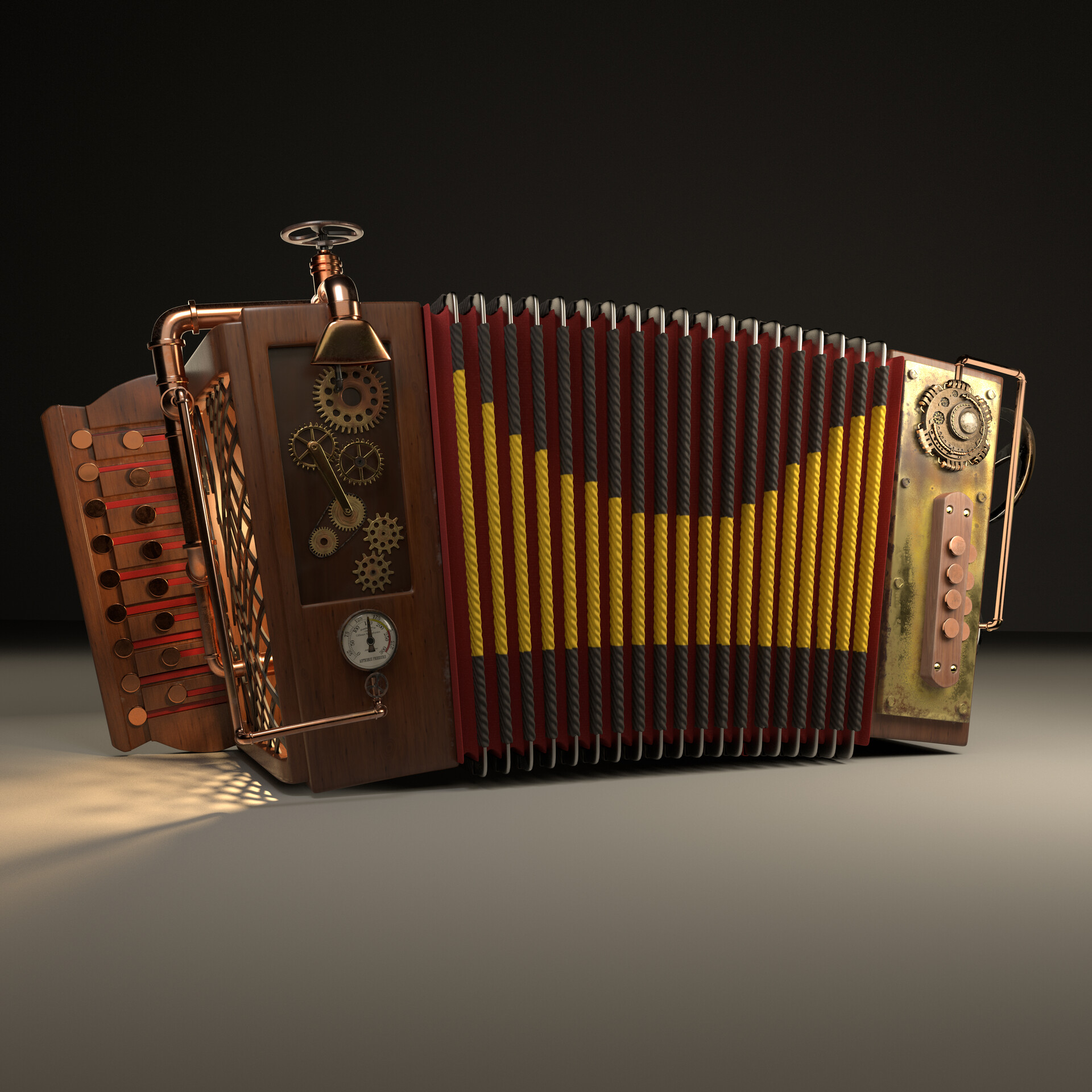This image showcases an antique, steampunk-style accordion resting on a gray surface with a completely black background, emphasizing its intricate details. The left console features a series of gears, cogs, and a gauge, contributing to its mechanical aesthetic. At the top of the left console, a brass valve resembling a garden hose spigot enhances the steampunk vibe. The bellows, extended in the middle, display a striking red interior with black and red exteriors arranged in a reverse bell curve pattern. Yellow highlights accentuate each rib of the bellows, creating a rhythmic visual flow. The right side of the accordion is distinguished by a brass handle and a dial with four buttons beneath it, against a background marked by a single prominent gear. The outer edges of the accordion are accentuated with brown hues and red lines, while the surface below exhibits a darker gray with lighter hints toward the right. Overall, the accordion's intricate design elements and steampunk motifs present a visually captivating and richly detailed instrument.